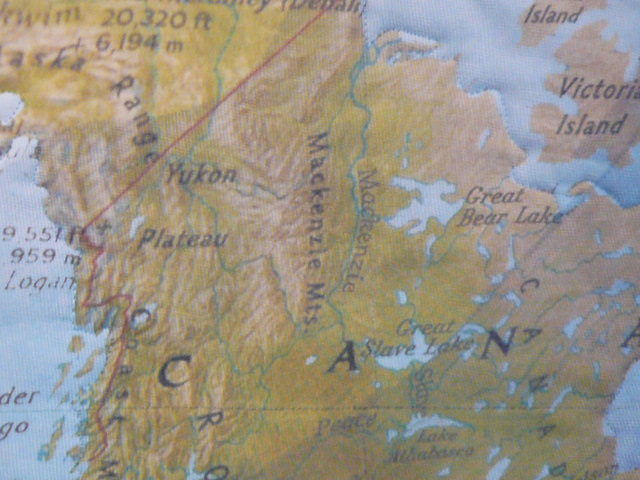This detailed image is a close-up geographical map featuring the western part of Canada, prominently showing regions such as the Yukon and Victoria Island, as well as parts of northern Alaska. The map includes notable geographical features like the Mackenzie Mountains, Great Bear Lake, Great Slave Lake, and the Yukon Plateau. Despite some text being unclear, the map displays topographical details such as various lakes, a plateau, and mountain ranges, highlighting the natural terrain with regions marked in browns and greens. The map is color-coded with blue representing the surrounding oceans. While the map does not focus on cities or states, emphasizing instead the physical landforms and altitudes, it artfully showcases the texture and natural formations of the land.